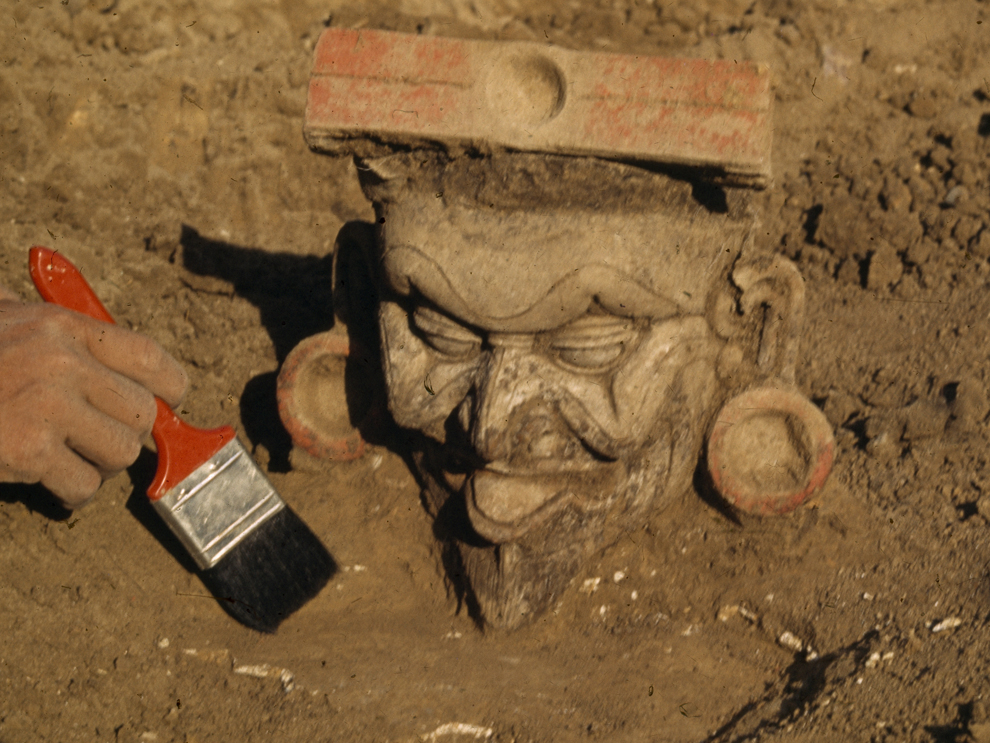In this color photograph taken in an outdoor setting, we see a detailed sand sculpture that appears to be modeled after a mythical figure, possibly a genie or a djinn. Central to the image is the sculpture’s intricately carved face, featuring a very long nose and a pointy chin. The mouth is open, and it is adorned with large earrings that resemble gauges. On top of the figure’s head is a reddish brick with a hole in the center. Surrounding the sculpture is a mixture of sand and gravel, some areas smooth and others disturbed as if recently dug up.

A hand is visible to the left of the sculpture, holding an orange-handled paintbrush with black bristles. The person appears to be carefully brushing away sand to further uncover the sculpture. This scene gives the impression that an archaeological excavation is underway, as the meticulous brushing suggests a focus on preserving delicate details. The earth around the sculpture is dark brown, indicating it might be slightly wet or muddy, adding to the authenticity of an excavation site.